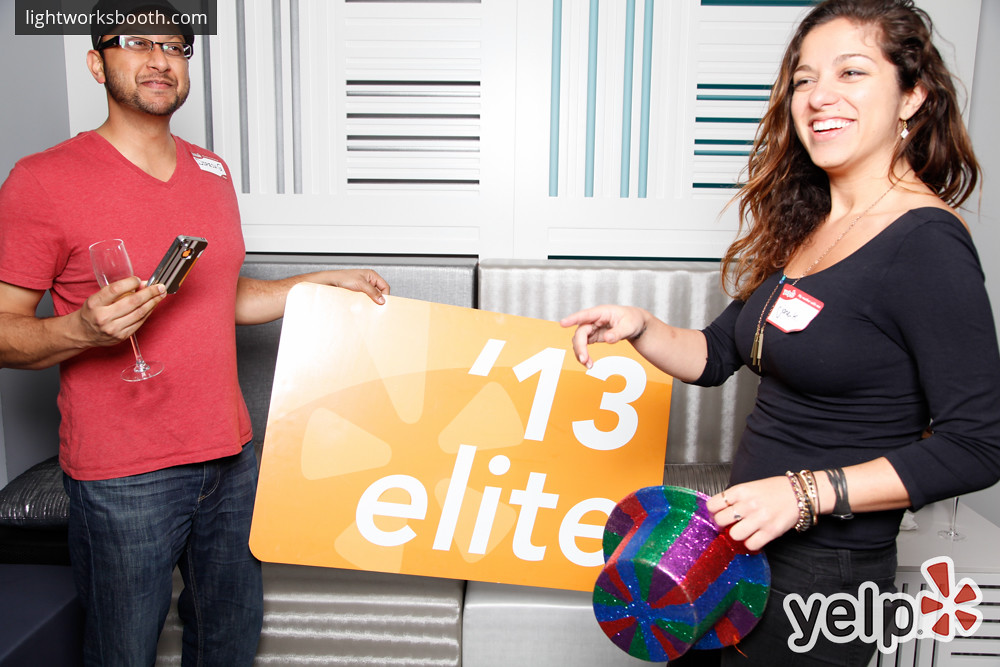The image depicts a man on the left and a woman on the right, standing in front of a white wall with blue stripes. The man has short hair, some facial hair, and wears black-framed glasses. He is dressed in a red v-neck t-shirt with a white name tag on his left shoulder and blue jeans. In his right hand, he holds a clear wine glass and an iPhone, while he also holds up a large sign that reads "13 Elite." The woman has long, wavy brown hair and is smiling. She wears a long-sleeve scoop neck black top with blue jeans. On her left wrist, she has multiple bracelets, and in her left hand, she holds a sparkly top hat with green, purple, blue, and red stripes. At the bottom right of the image, the Yelp logo with a red five-point star can be seen.